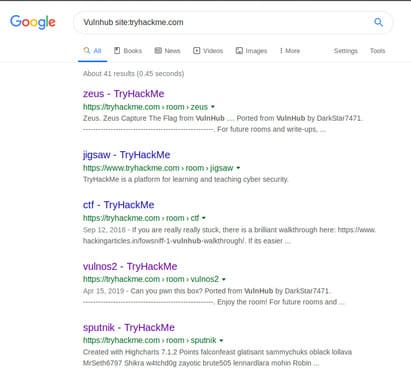The screenshot captures a Google search for "phonehub site:tryhackme.com." At the top of the page, it shows approximately 41 results fetched in 0.45 seconds. Below this, there are five website links, all related to TryHackMe. 

1. The first link, which is in purple indicating it has been visited, directs to "TryHackMe."
2. The second link, titled "Jigsaw TryHackMe" is in an indigo color, suggesting it has not been clicked.
3. The third link reads "CTF TryHackMe," also in indigo.
4. The fourth link, labeled "VulnOS 2 TryHackMe," is in purple, indicating it has been previously visited.
5. The final link, "Spitnik TryHackMe," is also in purple, indicating it too has been visited.